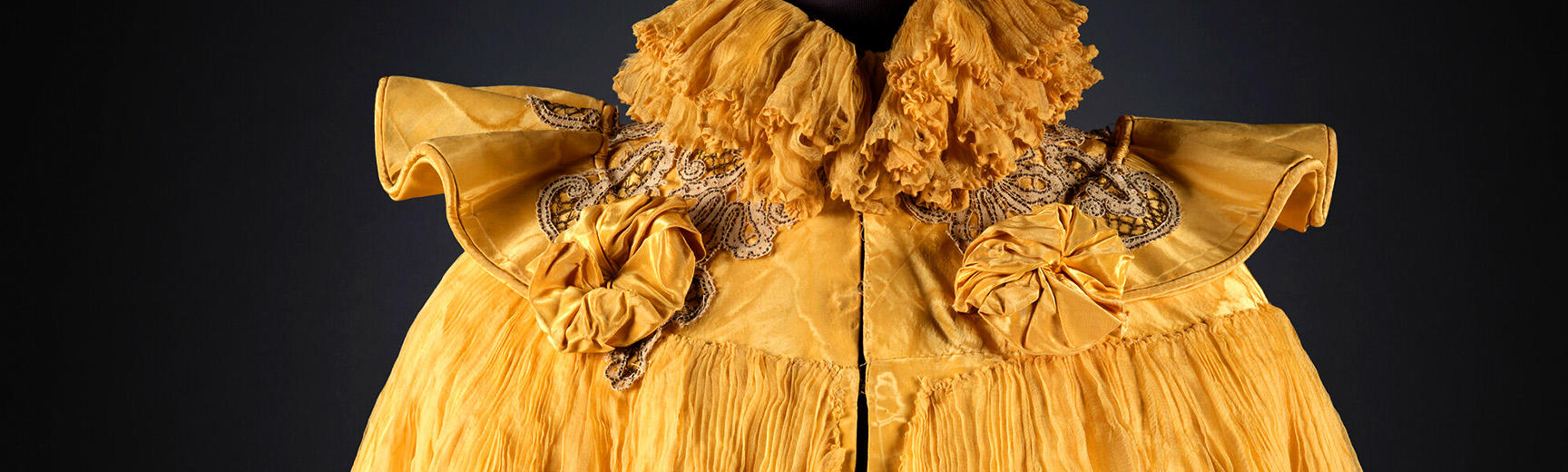The image features a zoomed-in view of the neckline of an elaborate, ornate garment that evokes Shakespearean costumes. The garment is predominantly a rich gold color, with a very ruffled, layered collar reminiscent of those worn in Shakespearean plays. Below the collar, there is a tan or gray lace-like design extending to the flared, ruffled shoulders, similar to a clown's costume. The fabric on the shoulders is wrinkled and extends outward, creating a theatrical look. Below these ruffled sections, there are darker, round areas resembling cloth donuts, with light reflecting off some spots. Further down, the garment transitions into lighter gold fabric with pleats and folds, leading towards a wide seam running down the middle, suggesting where it might open. The background is a deep, uninterrupted black, emphasizing the garment's intricate details.